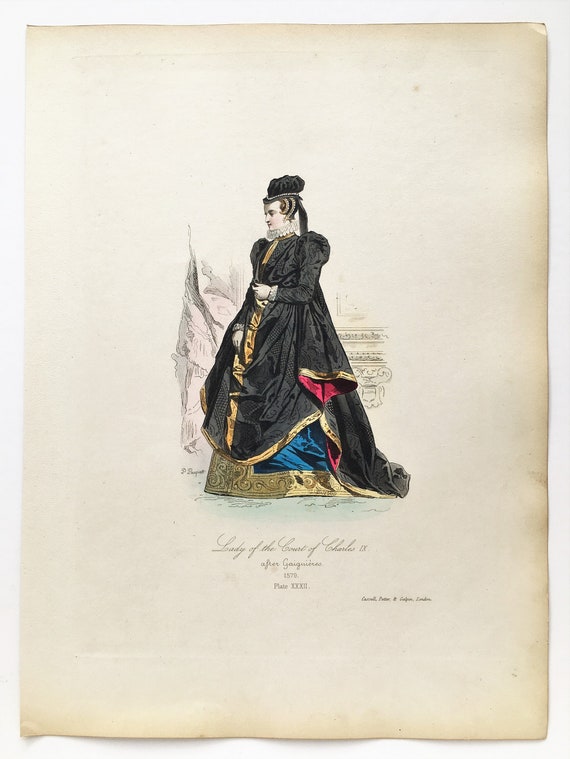This image depicts an old illustration on a piece of aged, browned paper. The central figure is a solemn-looking woman, identified as a "Lady of the Court of Charles 9," from the year 1579. She is adorned in a magnificent, elaborate outfit. Her black, satin dress features poofy sleeves, with gold trim around the hem, collar, and down the front. The dress is richly gathered and bunched, creating an opulent, voluminous effect. Inside the dress, a vibrant blue skirt trimmed with gold can be seen, with hints of red lining the interior. She wears a fluffy white, ruffled collar below her chin and matching white lace around the ends of her sleeves. Her accessories include a black, poofy hat with ribbons, pearl necklace, and curved gold pins in her hair. The background features indistinct wall-like elements with a light pink hue. The illustration is framed by empty space and contains indistinguishable words and names, although "Plate 32" and what appears to be the publisher's name are noted.